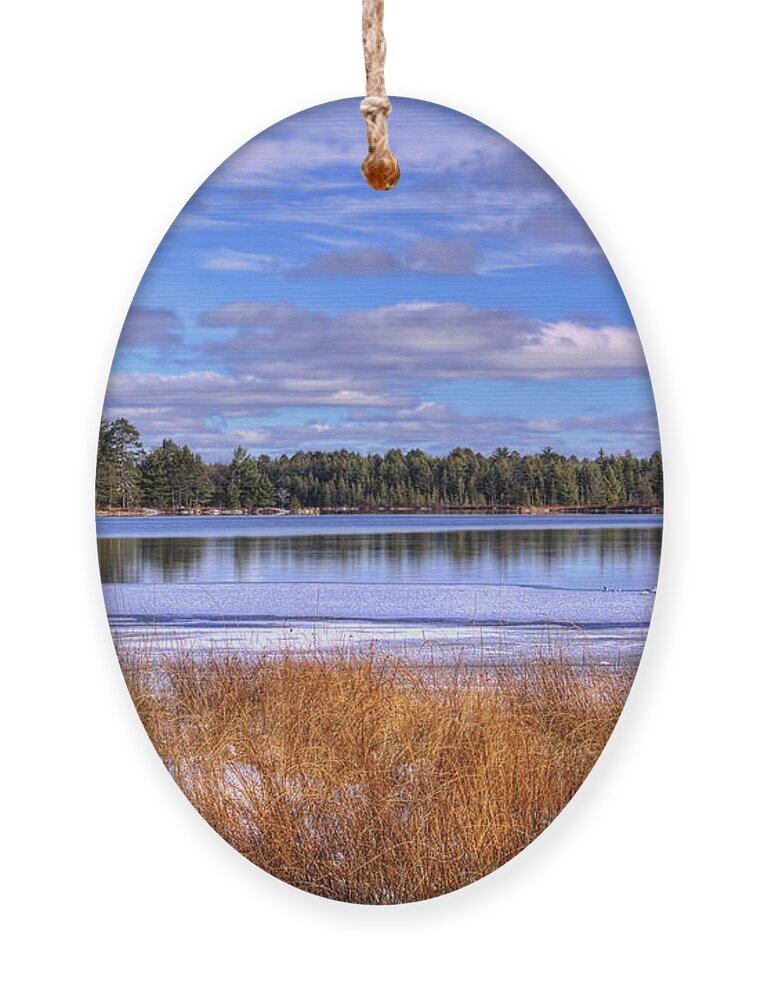This decoration features an oval-shaped ornament suspended from a light brown rope, resembling a piece of wall art or a pendant. The scene depicted within the oval comprises a serene winter landscape. The foreground is filled with sparse, golden-brown, dried grasses lightly dusted with snow. Stretching out behind the grass, the water of a lake reflects the surrounding environment, showing gentle ripples that capture the image of the tree line and the sky above. The lake's deep blue hue contrasts with the icy patches near the shore. Beyond the water lies a dense assembly of evergreen and pine trees, typical of a winter forest, their reflection shimmering in the lake. Above this idyllic scene, a vast, bright blue sky is scattered with pillowy clouds in various shades from white to light gray, creating a picturesque and calm atmosphere. The overall composition, reminiscent of a framed painting, provides a detailed and peaceful vista of nature in the colder months.